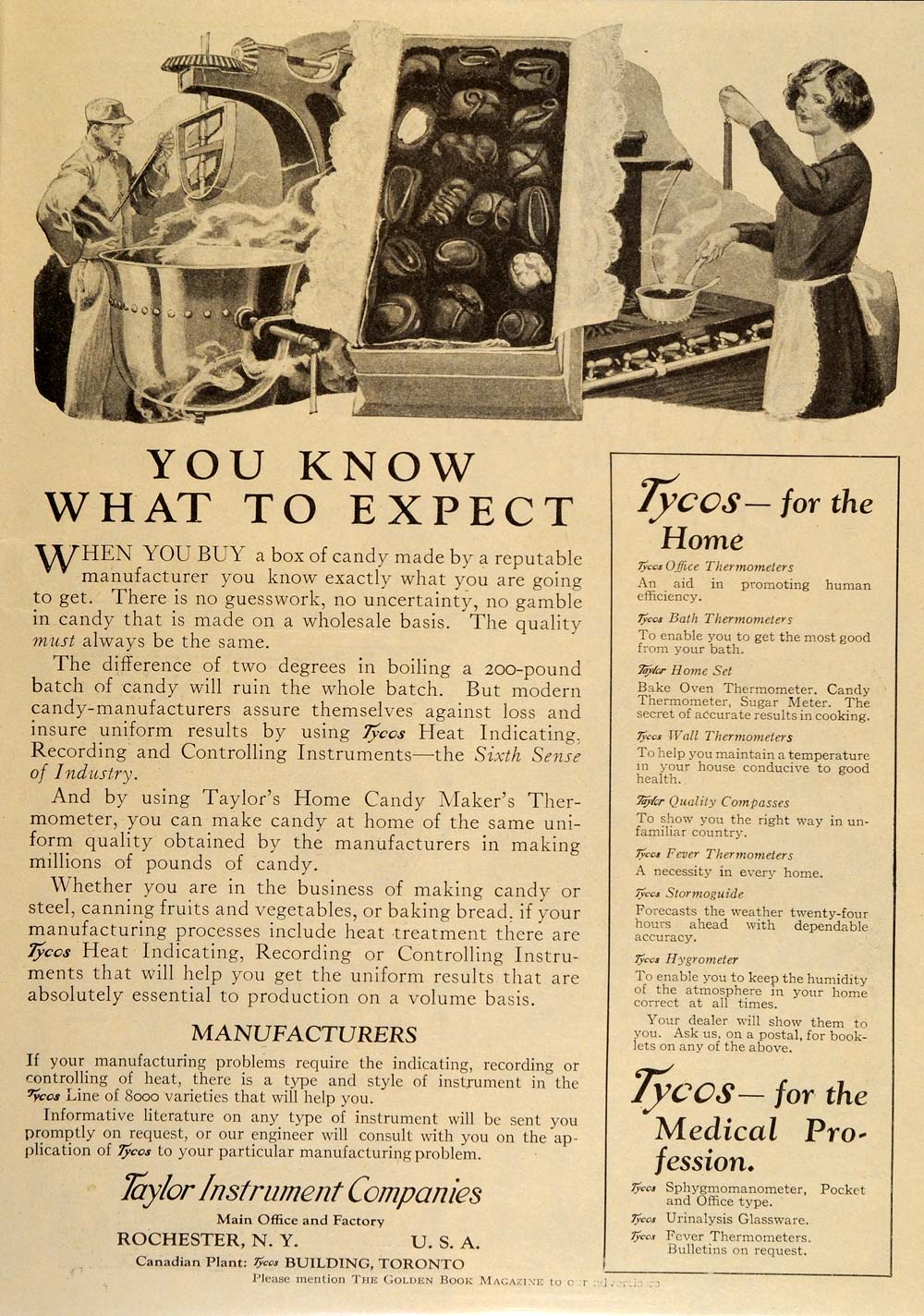This vintage print advertisement, displayed on an aged ivory background, showcases detailed black-and-white illustrations at the top. On the left, a man operates a colossal stand mixer, diligently checking the temperature of the substance inside. In the center, an open box of assorted chocolates is elegantly arranged, with a doily partially covering it to reveal the variety of confections. On the right, a woman, donned in a dress and white apron, attentively monitors the temperature of a pot on a gas stove, with visible steam rising. Beneath these captivating images, the text proclaims, "You know what to expect," emphasizing the importance of precise temperature control in candy making. The ad is credited to the Taylor Instrument Companies, located in Rochester, New York, and mentions their offerings, including "Tycos for the home" and "Tycos for the medical profession," highlighting their extensive range of thermometers.